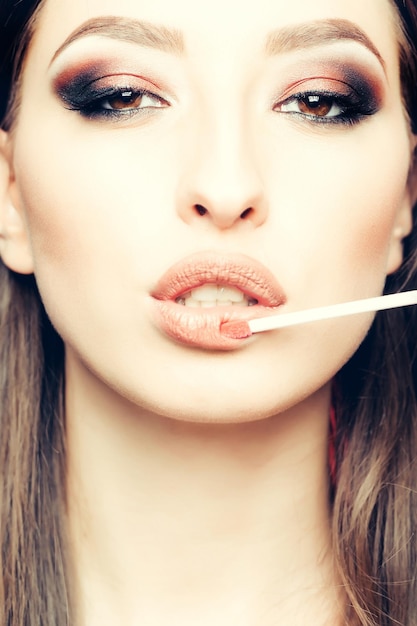This is a close-up image of a Caucasian model with brown eyes and pronounced facial features. The focus is primarily on her face, revealing her thick, colored-in eyebrows and black smoky eyes accentuated with copper eyeshadow and black eyeliner beneath. Her eye makeup is bold, featuring elements of red and black hues. Her lips, pouted and slightly parted, display a glimpse of her white teeth. A white applicator with a peachy nude or red color, resembling either a lipstick brush or a matchstick, is touching her bottom lip. She has long, straight dark brown hair and a smooth, porcelain-like neck. Only part of her forehead is visible, highlighting the intimate, detailed nature of the close-up shot. Her expression and the placement of the applicator suggest a sense of poised aesthetic focus.